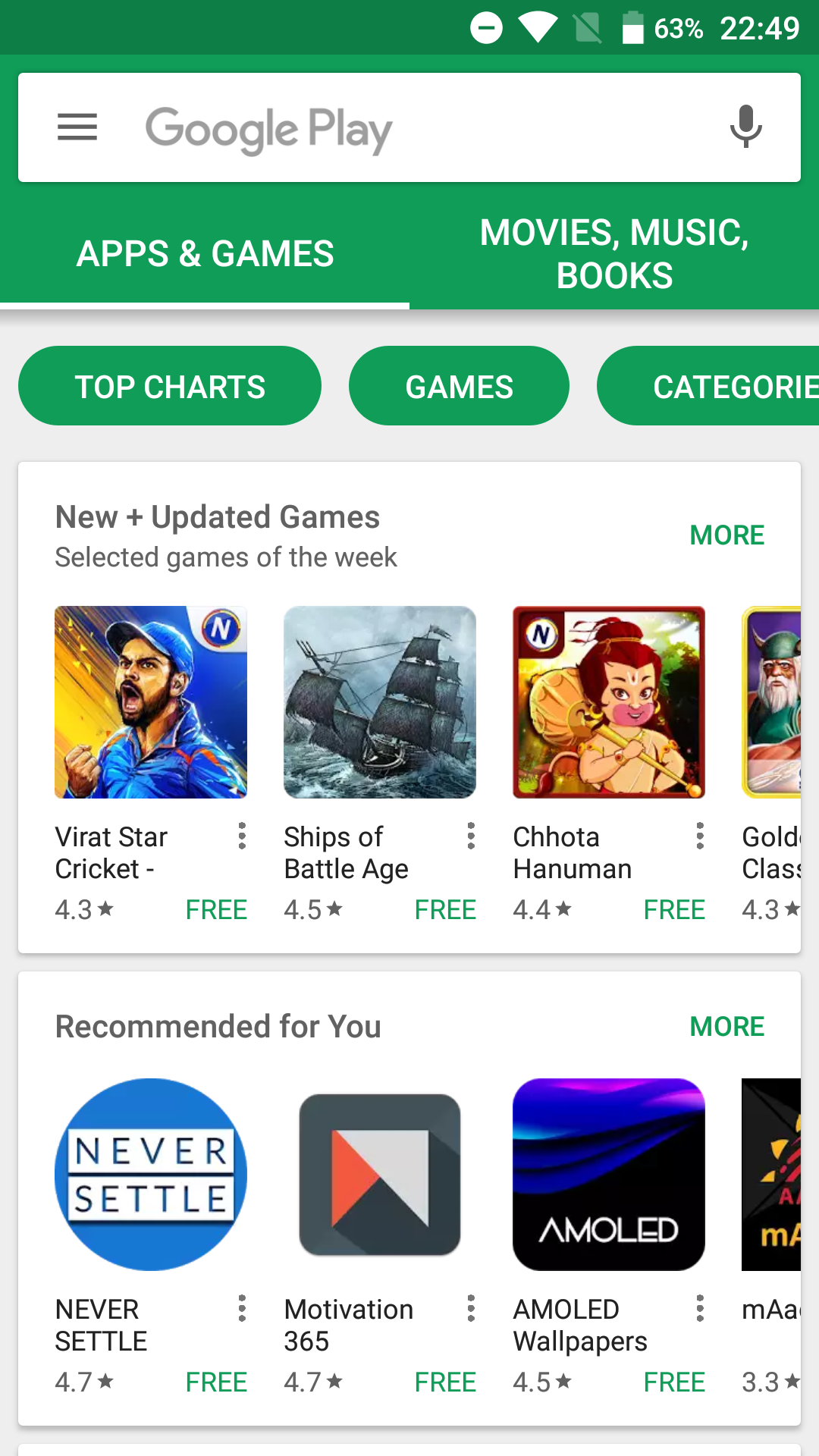This portrait-oriented, color screenshot captures the display of a smartphone at 22:49, with a battery life of 62% and full Wi-Fi connectivity. The screen shows the Google Play Store, an app used for downloading and accessing various other apps, both free and paid. At the top, a green banner houses a white search field for easy app lookup.

Below the banner, there are two primary tabs: "Apps & Games" and "Movies, Music, Books." Scrolling down, the screen showcases a variety of featured apps. The "New & Updated Games" section highlights titles such as "Viral Start Cricket," "Ships of Battle: Age of Pirates," and "Chhota Hanuman," displaying a mix of gaming genres without a clear thematic link.

Further down, the "Recommended for You" section appears, featuring apps like "Never Settle Motivation," and "AMOLED Wallpapers," which cater more towards personal improvement and customization. The screenshot provides a detailed glimpse into the user's app browsing experience on the Google Play Store, capturing an eclectic mix of gaming and motivational content.